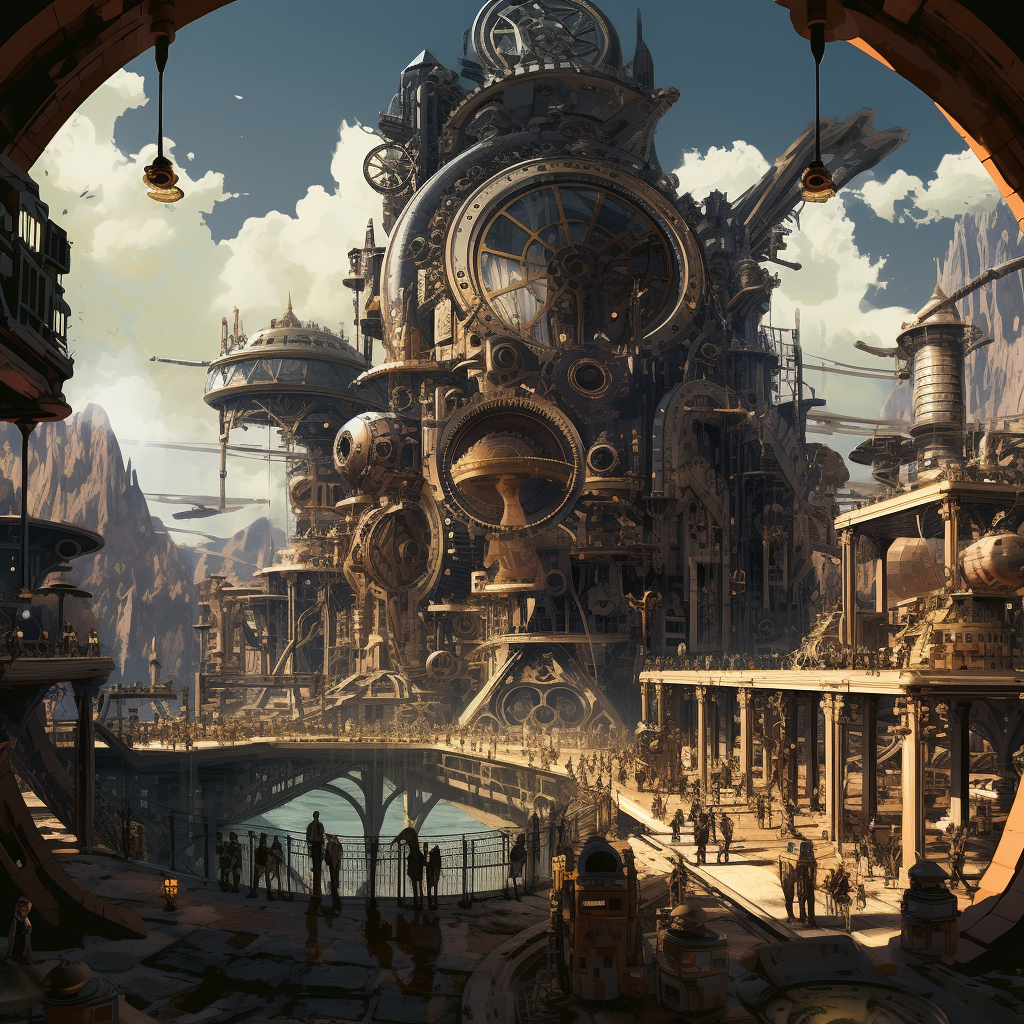The image depicts a highly detailed, 3D computer-generated illustration of a massive steampunk-inspired city, lying on the edge of an ocean or sea. The scene is framed by a large, oval opening that gives a panoramic view of the intricate cityscape. At the forefront, a spacious balcony and walkway lead towards a monumental central building. This colossal structure is a marvel of steampunk engineering, composed of enormous gears, circular glass windows, and various industrial components arranged in a makeshift yet meticulously detailed manner.

The city is predominantly brown in color, evoking the quintessential steampunk aesthetic. Intricate machinery, including a distinctive rocket-shaped apparatus, is seen to the right. Identical light fixtures hang in the upper left and right corners, casting a soft glow over the futuristic public square filled with silhouettes of people milling about.

The day is bright with sunlight streaming from the left, casting shadows and illuminating the scene. The sky is mostly cloud-covered with patches of blue peeking through. Mountains rise in the background, adding depth to the landscape. Overall, the image skillfully combines elements of fantasy and science fiction to create an immersive steampunk metropolis.